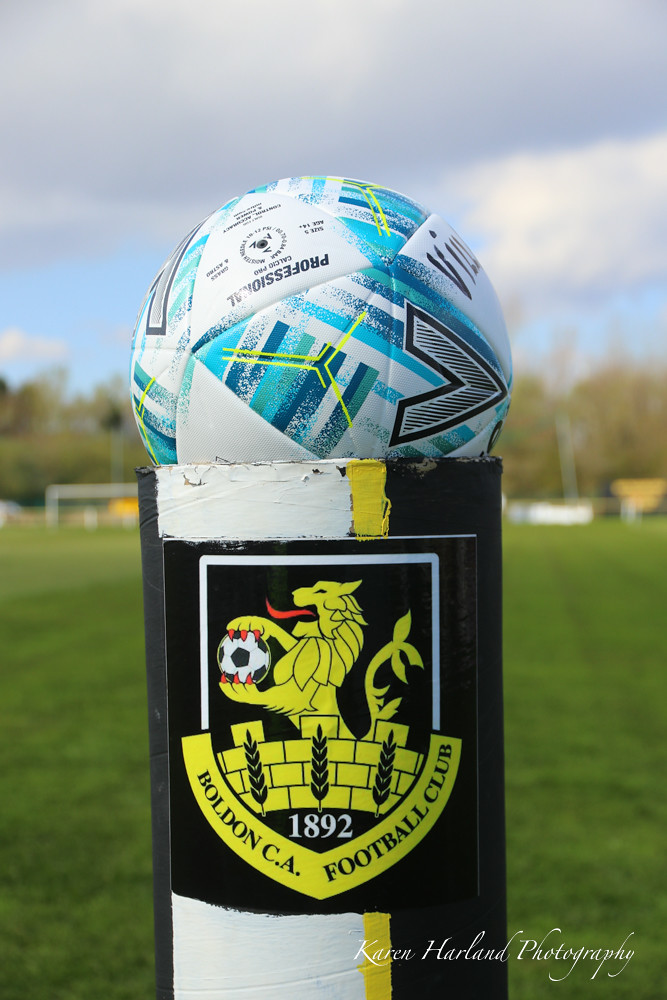The photograph captures an outdoor soccer field bathed in a bright, sunny day with a vibrant blue sky dotted with white and gray clouds. The background, though out of focus, features a lush green grass field stretching into the distance, with a distinct soccer goal about 60 to 70 yards away. Beyond the goal, there is a tree line, suggesting a wooded area or trees just outside the stadium.

Dominating the foreground is a striking trophy set against this picturesque backdrop. The trophy consists of a black cylindrical podium adorned with alternating white and yellow stripes. Prominently displayed on the front of the podium is the regal logo of Bolden CA Football Club, featuring a lion holding a soccer ball, inscribed with the founding year "1892". The logo sits above a white and yellow patch that wraps around the top of the cylinder.

Perched on top of this pedestal is a professional soccer ball, decorated with alternating patterns of white, blue, and yellow, and marked by a repeating V motif. The entire setup is enhanced with the professional touch of "Karen Harland Photography" elegantly scripted in the bottom right-hand corner of the image.